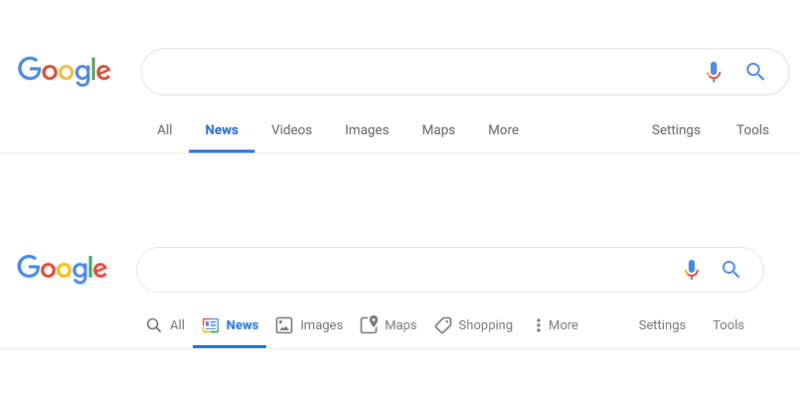At the top left corner of the image, the iconic Google logo is displayed, featuring its recognizable colors: blue, red, yellow, and green. Alongside it extends a long, rectangular search bar. At the end of the search bar, there is a blue microphone icon followed by a magnifying glass icon. Below this, a navigation bar includes the words "All," "News" (highlighted in blue and underlined), "Videos," "Images," "Maps," "More," and, separated by an approximate four-inch gap, "Settings" and "Tools."

Repeating lower in the image, the Google logo appears again with the same search bar, complete with the blue microphone and magnifying glass icons. Under this search bar, there is another magnifying glass icon to the left, followed by the phrasing "All" in gray text, "News" (again highlighted in blue and underlined), and a multicolored square representing Google. Following these are links for "Images," "Maps," and a small tag labeled "Shopping." Adjacent to these options are three vertical dots for additional settings, "More," and the options "Settings" and "Tools" in gray text.

This detailed layout highlights the components of a typical Google search results page, focusing on the navigation and interactive elements available to the user.